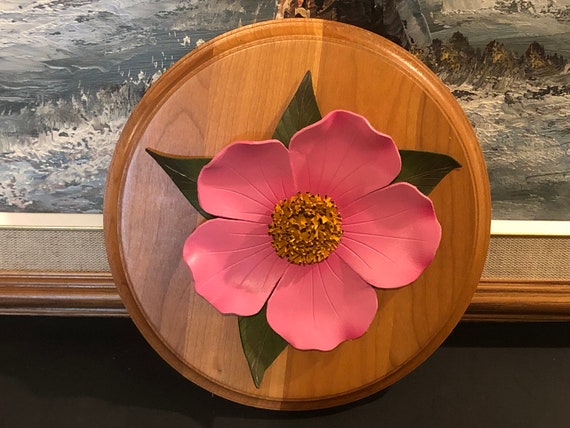The photograph captures a detailed scene with multiple elements. In the foreground, there's a well-polished, circular wooden board on which sits a detailed sculpture of a flower. This flower sculpture, likely made of plastic, features five pink and white petals, a yellow stamen, and four rectangular green leaves around its base. The circular wooden board appears to be placed on a black or dark brown surface. In the background, a larger landscape painting with a golden-brown wooden frame is visible. The painting itself depicts an oceanic scene with waves, some rocks or cliffs, and mountains. The painting's frame has a thin white border, and although much of the painting is obscured by the circular board, the glimpses of the sea and mountainous landscape add depth to the scene. The entire setup looks meticulously arranged, combining natural-themed art and crafted elements in a cohesive display.